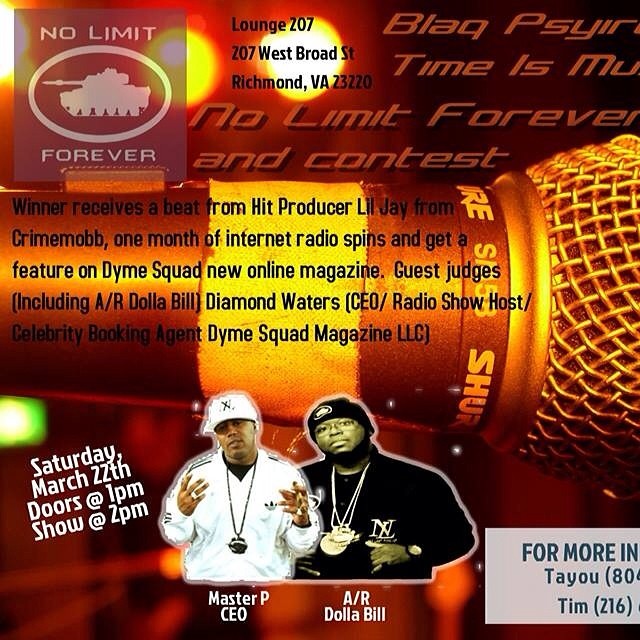This is a detailed and comprehensive caption from the gathered information:

---

A vibrant flyer announces a music performance with exciting attractions. The event is scheduled for Saturday, March 22nd, with doors opening at 1 PM and the show starting at 2 PM, prominently displayed in white text on the lower left corner. The background features a dynamic palette of red, orange, black, and yellow hues creating an eye-catching backdrop. A large, horizontally positioned microphone image dominates the center, adorned with various text written over it.

In the upper left-hand corner, the logo "No Limit Forever" appears with a military vehicle, while the top of the flyer reads "Lounge 207, 207 West Broad Street, Richmond, VA, 23220" in black text. Further details include the phrase "Black Sire, Time is Moo," although some parts appear to be partially obscured.

The flyer highlights that the winner of the contest will receive a beat from hit producer Lil' J from Crime Mob, one month of internet radio spins, and a feature in the new online magazine Dime Squad. Esteemed guest judges for the event include A.R. Dolla Bill, Diamond Waters, CEO, Radio Talk show host, celebrity booking agent, and Dime Squad Magazine LLC.

Prominent images of two key figures are at the bottom: Master P, the CEO, dressed in all white with a matching white hat, and A.R. Dolla Bill, dressed in all black with a matching hat. Additional information appears to the right, including a note that says "More Info" followed by partially visible contact details.

---

This caption combines the overlaps and key points from all provided descriptions to create a detailed and cohesive summary of the flyer.